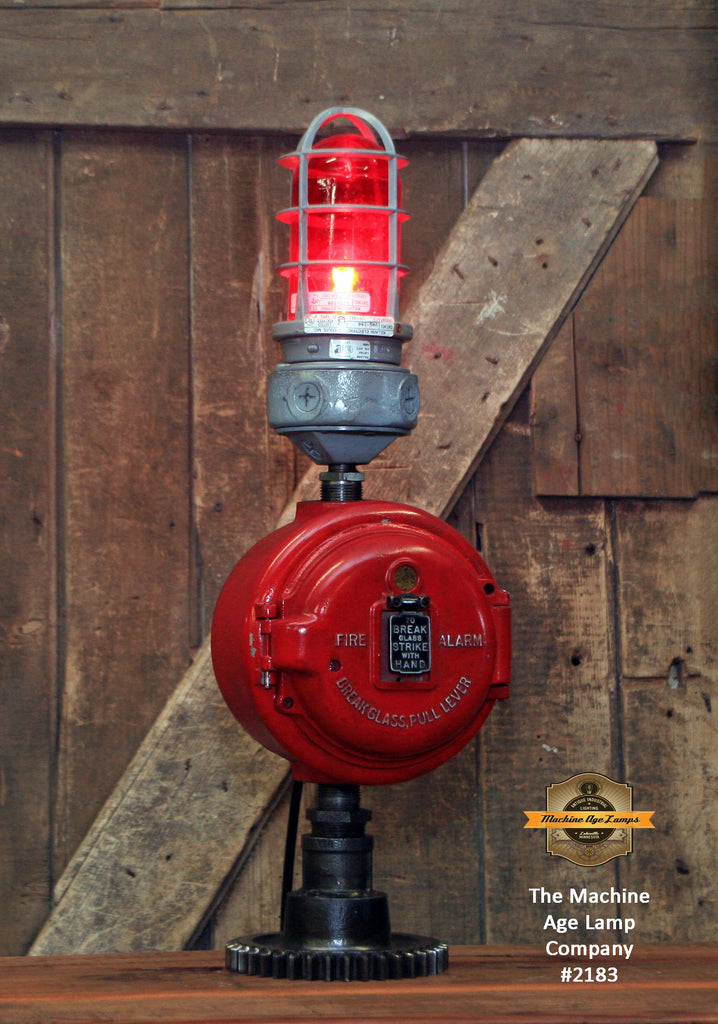This is a detailed close-up photograph of an old fire alarm sitting on a wooden shelf against a wooden wall. The device features a distinctive red, circular body made of steel, with a black, gear-like base that extends upward into a black tube connecting to the alarm. On top of the alarm, there is a red bulb light that can flash, reminiscent of a police siren. The front of the device has a round meter-like face with instructions in small letters: "FIRE ALARM - Break glass - Pull lever". In the middle of the alarm, it says "Break glass - Strike with hand." The device also has a door that must be opened to access the pull lever. In the lower right corner, the words "The Machine Age Lamp Company No. 2183" are printed, identifying the maker. This vintage piece combines both industrial charm and practical function.